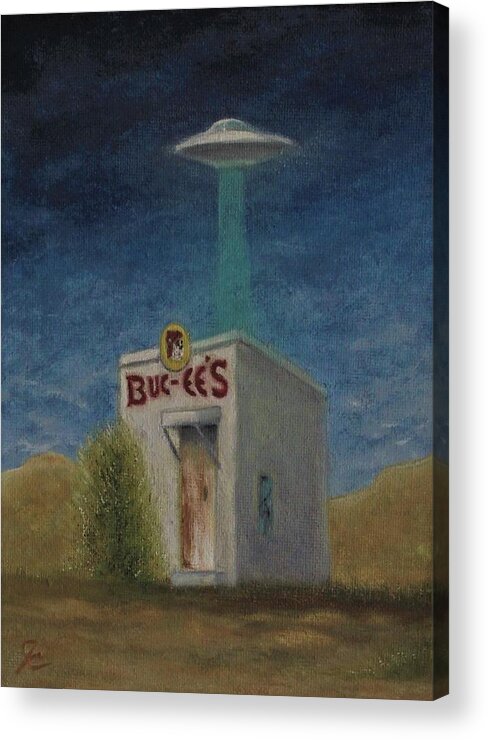This artwork features a vividly detailed scene of a small establishment named "Buc-ee's," which resembles a quaint, outdoor restroom or outhouse, set against a dramatic, dark blue night sky that lightens towards the horizon. The building's off-white facade is adorned with the "Buc-ee's" logo, spelled in red letters outlined in yellow, along with a mascot depicted as a bulldog (or possibly a chipmunk) wearing a beanie. This rustic structure includes a brown wooden door shaded by a small overhang, a window or poster on the side, and a green bush in front. Above the structure hovers a classic UFO, silvery white with a bluish-green beam projecting downwards as if poised to abduct the tiny building. The surrounding terrain appears to be rolling hills of perhaps dead grass, lending a desolate, New Mexico-like atmosphere to the scene, further accentuated by a lonely tree on the left side of the building. This evocative painting combines elements of whimsy and mystery, capturing the imagination with its surreal blend of everyday Americana and extraterrestrial intrigue.